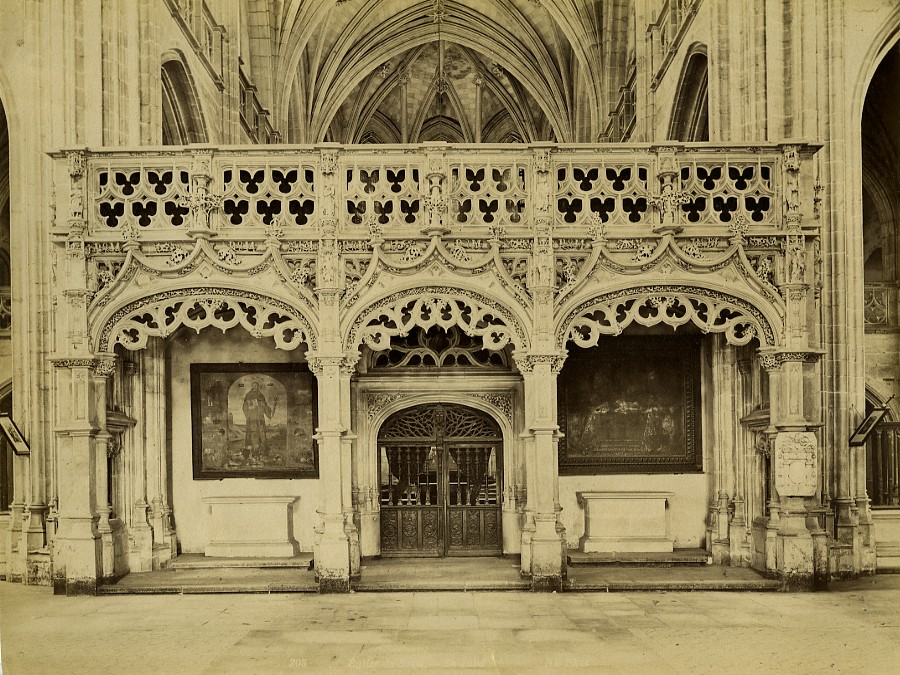This detailed black-and-white photograph, approximately 6 inches wide and 4 inches high, captures the interior of a gothic, likely orthodox, church or cathedral. The foreground is covered with grey marble tiles or cement pavestones. In the midground, a large, ornate balcony with a delicate hand railing is visible on the second floor, supported by massive stone columns. Below the balcony are three grand, arched doorways; the central doorway, distinguished by a black door, is flanked by two arches housing recessed artworks. The left artwork appears to depict a solitary figure, while the right one possibly shows two figures, though their details remain ambiguous due to the photograph's darkness. The walls, adorned with placards, stretch upwards to a vaulted or domed ceiling, elaborately decorated with spires and ecclesiastical imagery. Two additional doorways and a placard are partially visible at the far edges of the frame, enhancing the image's intricate stone craftsmanship and historical ambiance.